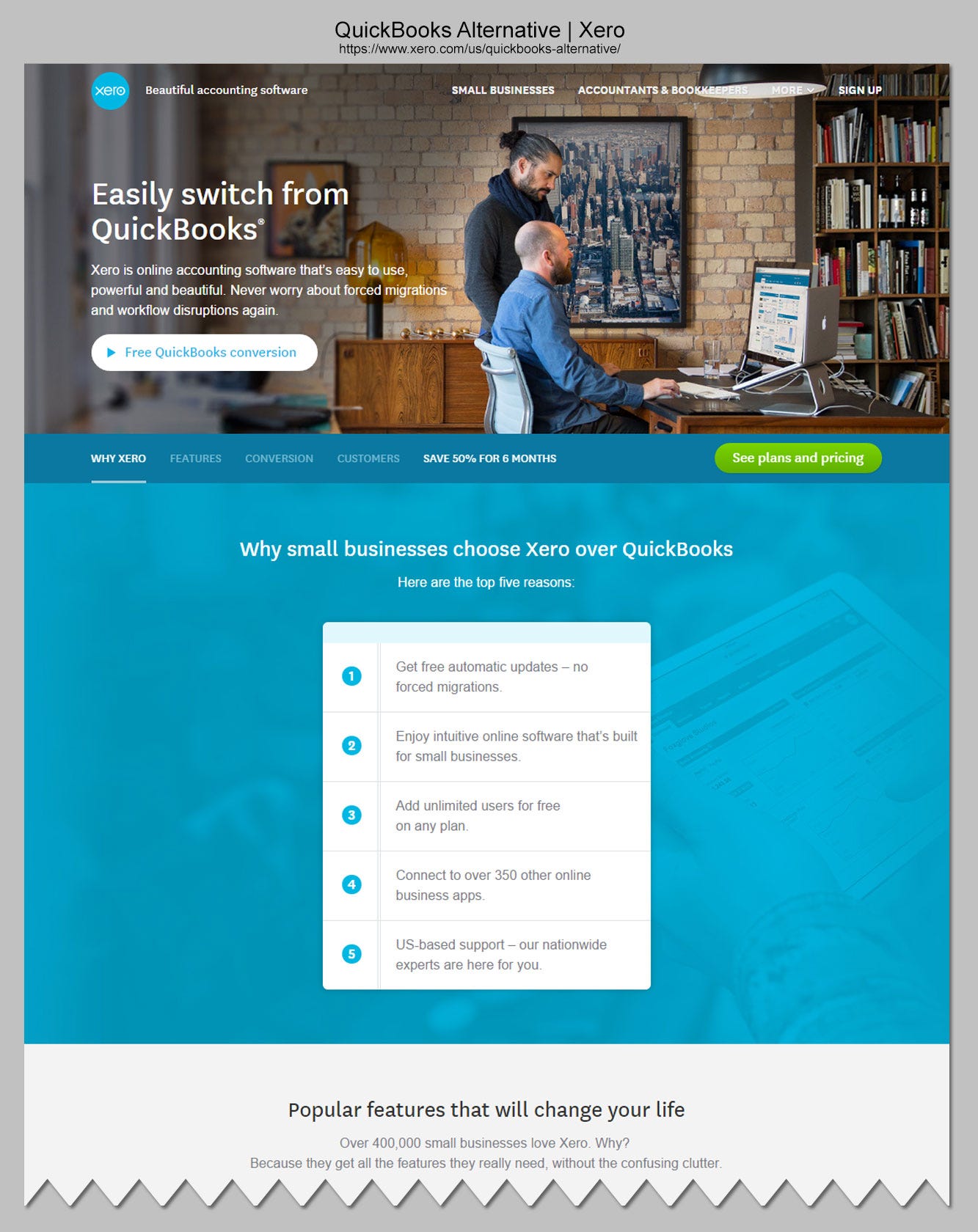### Detailed Descriptive Caption:

The image presents a comprehensive promotional graphic for an alternative to QuickBooks. The backdrop is a medium gray tone, providing a neutral base that allows the content to stand out. At the top center of the image, bold black text reads "QuickBooks alternative," with "QuickBooks" capitalized correctly with a capital Q and B.

Beneath this title, there's a horizontal line followed by "Zero" written with a capital X and an arrow indicating forward motion. A web address is listed underneath this.

Descending further, the image features a detailed graphic depicting two people inside a home. The setting includes a library-like bookshelf filled with numerous books. The individuals are positioned at a desk with a computer; one person is standing while the other is seated.

Accompanying this graphic, text emphasizes the ease of switching from QuickBooks: "Easily switch from QuickBooks. Zero's online accounting software is easy to use, powerful, and beautiful. Never worry about forced migrations and workflow disruptions again."

Highlighted in a white banner or tab, blue text announces "Free QuickBooks conversion."

At the bottom of the image, a section with a blue background states in white, underlined text, "Why Zero?" This is followed by several compelling features in white text: 
- Customers save 50% for six months
- Free QuickBooks conversion

Additionally, a green tab prompts viewers with "See plans and pricing."

Another blue backdrop further outlines why small businesses prefer Zero over QuickBooks, listing five top reasons:
1. Free automatic updates
2. No forced migrations
3. Intuitive online software built for small businesses
4. Unlimited users are free on any plan
5. Convert to over 350 other online business apps

The graphic concludes by highlighting "US-based support: Our nationwide experts are here for you," along with a note about "Popular features that will change your life."